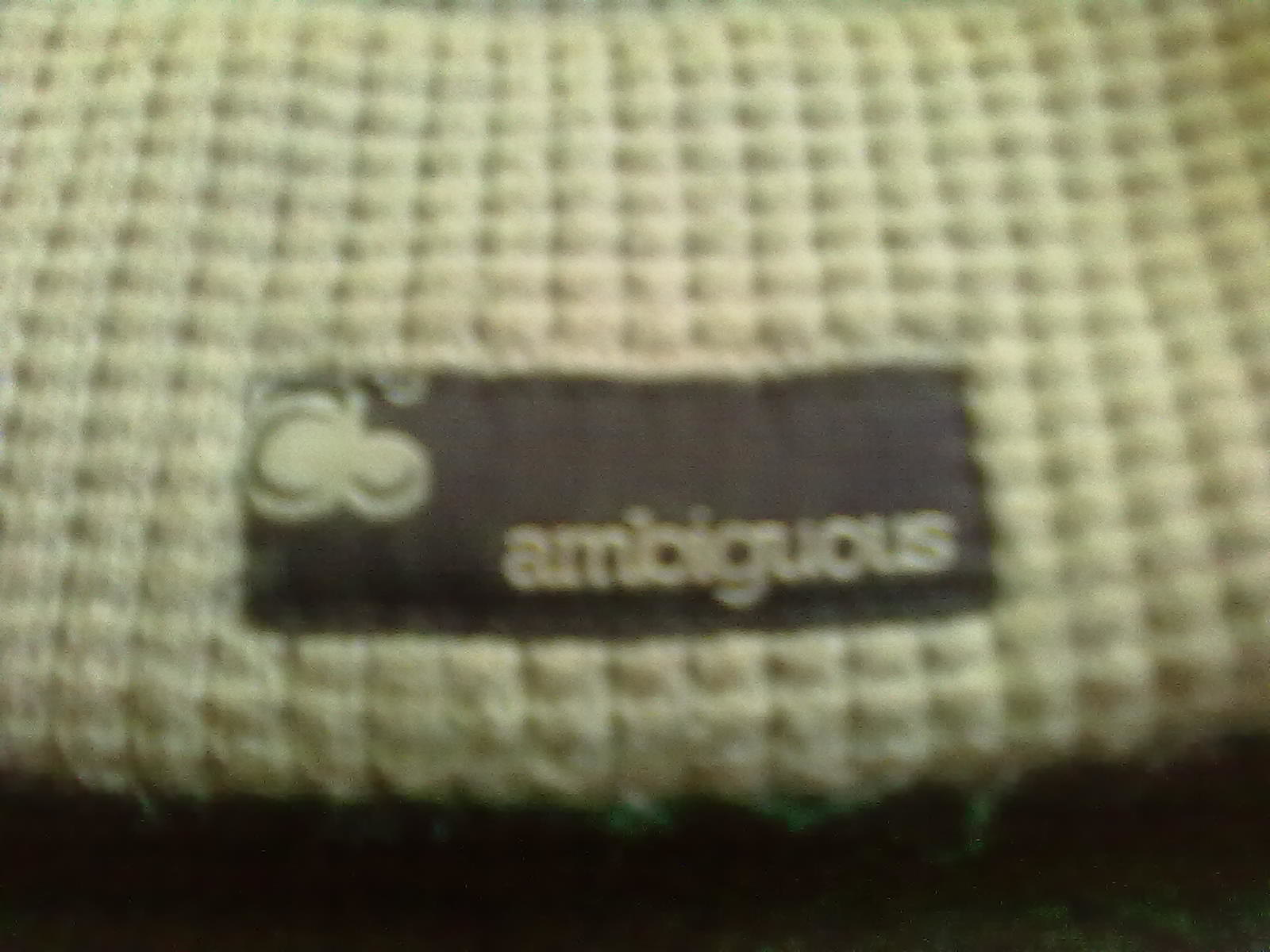The image portrays a waffle weave fabric, possibly a hand towel or a thin blanket, in a pale yellow hue. The material, distinguished by its textured pattern, suggests it may be more substantial than a typical hand towel. The photograph is taken in a dimly lit environment, resulting in a somewhat blurry and dark composition. Positioned centrally on the fabric is a black label, prominently featuring the word "ambiguous." The label includes a logo situated in the upper left corner, both the lettering and logo matching the fabric's pale yellow color, blending subtly into the material. The overall ambiance of the image is shadowy, with a black foreground enhancing the sense of obscurity.